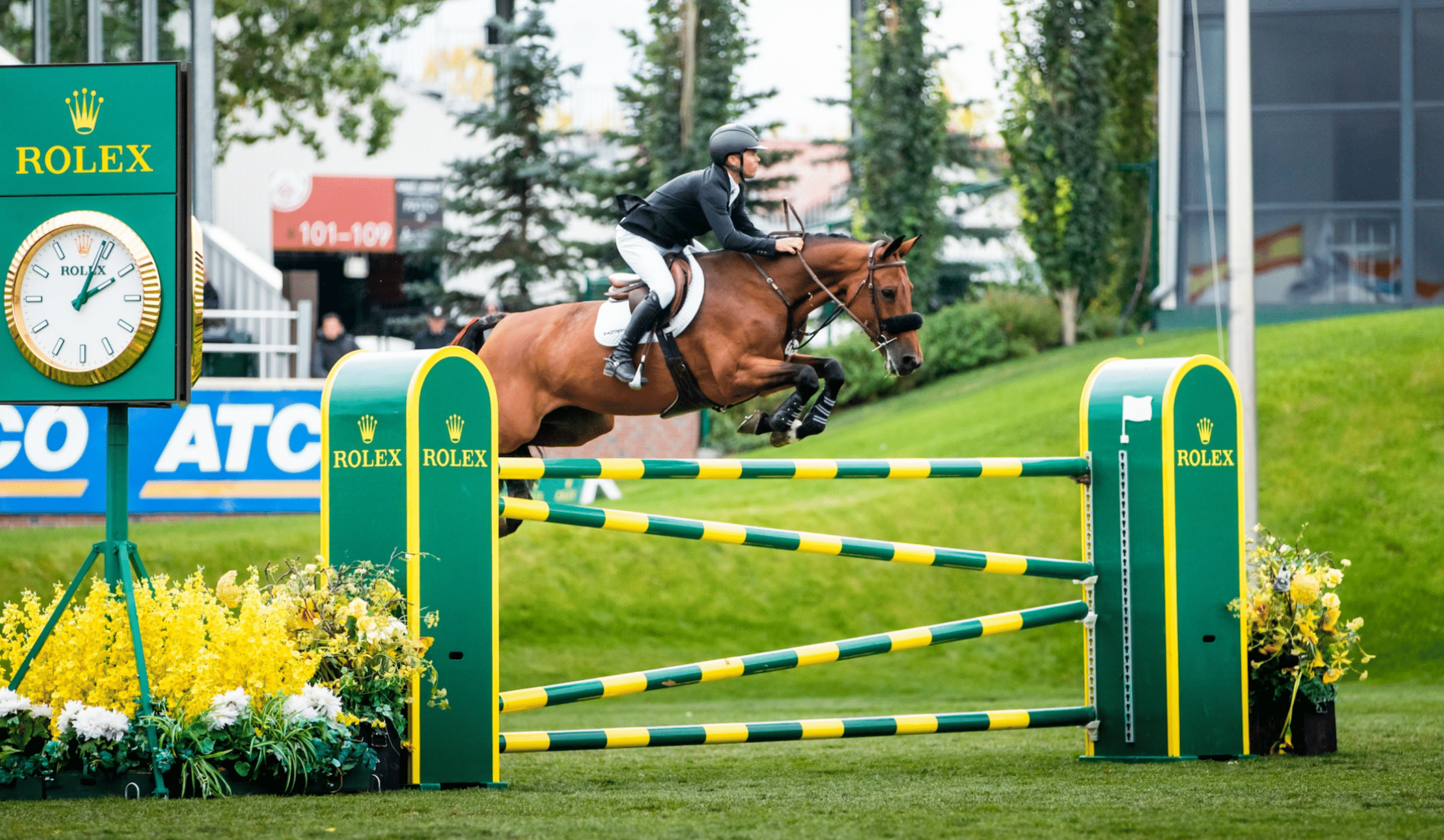In this outdoor photograph, a jockey in a traditional black and white outfit with a black helmet is captured mid-jump on a brown horse during an equestrian competition. The setting features a vividly detailed obstacle course sponsored by Rolex. The horse and rider are seen clearing a green and yellow striped gate flanked by two posts, both prominently displaying the Rolex logo in yellow letters. Below a large green sign with the Rolex name, a clock further emphasizes the brand's sponsorship. The background showcases a lush green grassy hill dotted with trees, adding depth to the scene. Nearby, there is a ticketing booth marked "101-109" and a building in the top right corner. Bright yellow flowers around the fence add a touch of color to the action-packed scene.